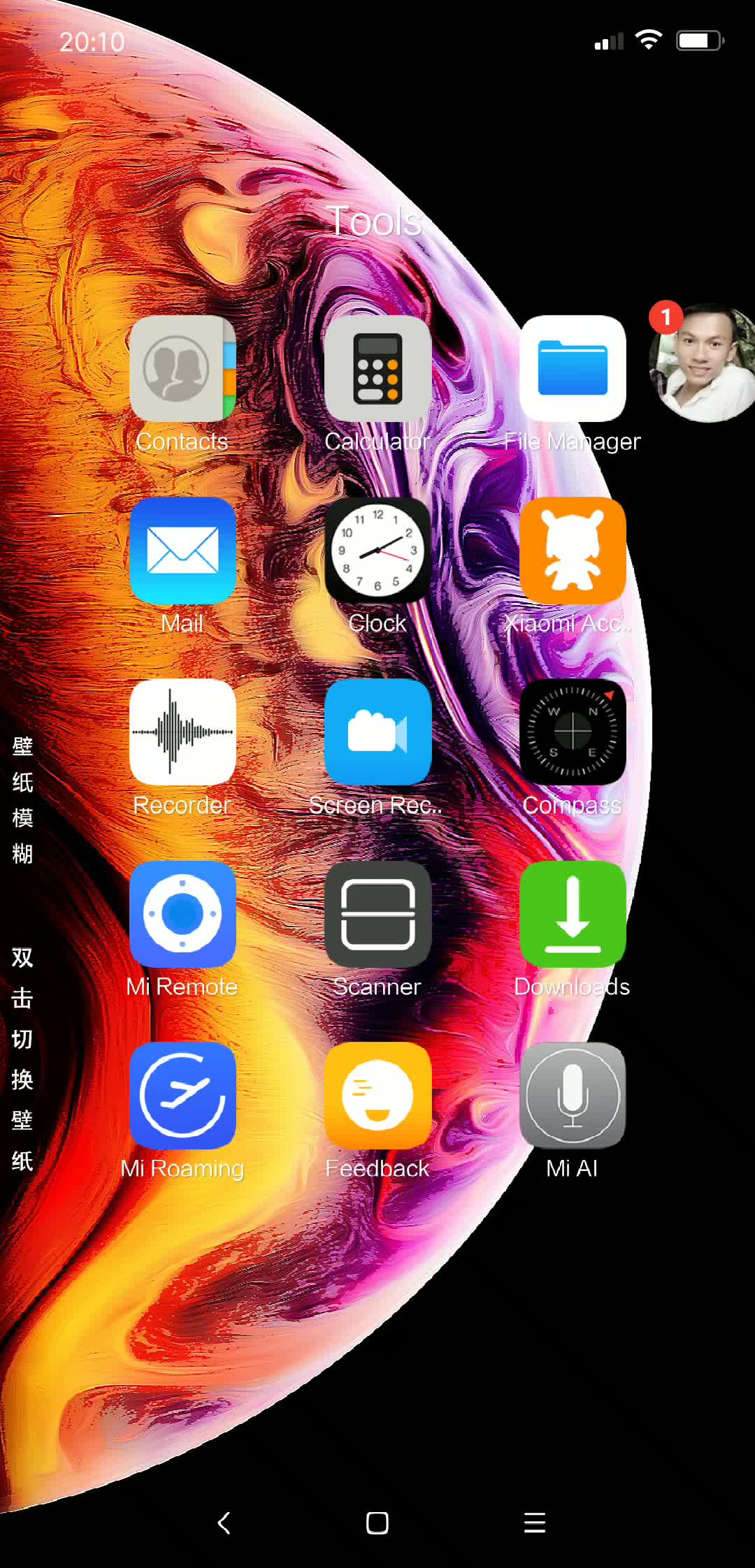The image is a detailed screenshot of a smartphone's home screen, specifically showing a folder labeled "Tools." The phone appears to be a new Samsung model, characterized by its long, rectangular shape and sharp edges. However, there's a momentary confusion suggesting it might be an iPhone due to familiar icon design, though ultimately confirmed as a Samsung device.

The background is space-themed, predominantly featuring a black backdrop with colorful, swirling marble-like planets in purple, orange, and red dominating the screen. The focus is on the opened "Tools" folder, displaying multiple app icons including Contacts, Calendar, Mail, Clock, Recorder, Me Roaming, Me AI, Downloads, and Compass.

A small, circular profile picture is located next to the app icons, depicting an Asian man wearing a white shirt, indicating the phone belongs to him.